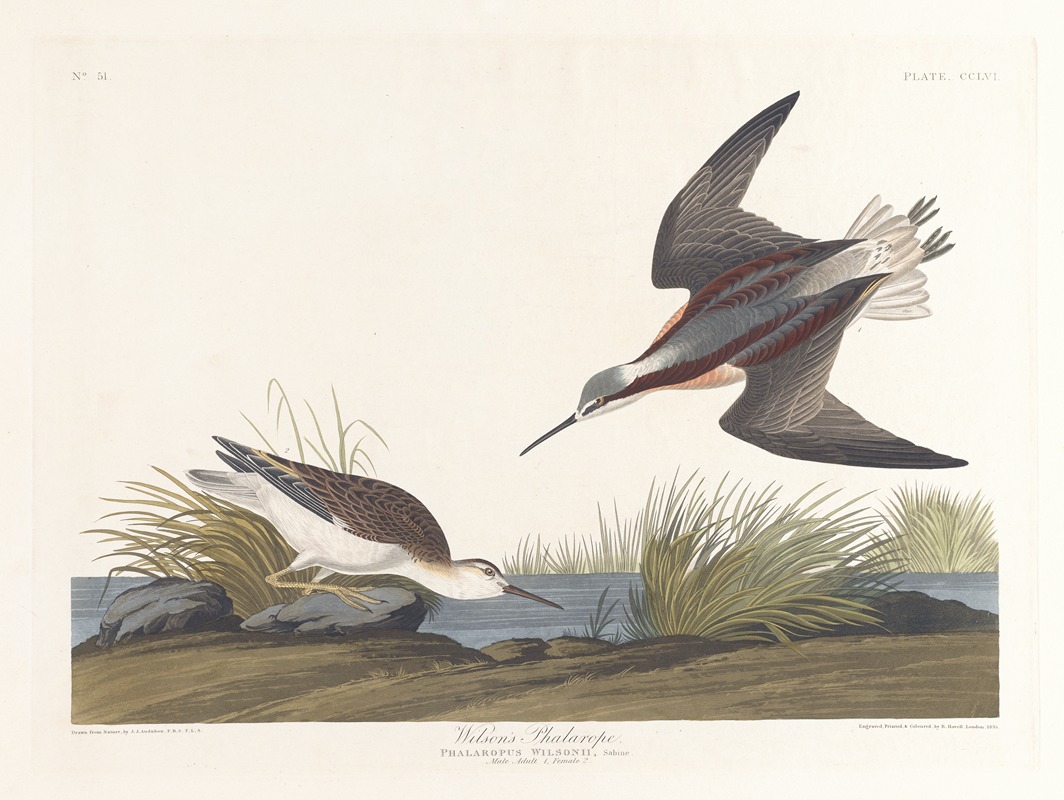This image is a hand-drawn painting of birds that exudes a vintage, almost antique appearance, akin to something one might find in an old book. The artwork, rendered in faded, earthy pastels, rests on a beige-ish background hinting at signs of age. In the foreground, the scene captures a shore's edge adorned with dirt, gray rocks, and small patches of green grass as blue water stretches out to the horizon.

The left side of the painting depicts a bird perched on a gray rock, leaning to drink from the water. This bird features brown feathers on top, a white belly, and yellow legs. The intricate details of its plumage include subtle hints of blue and white, with a sharp, pointed beak.

To the right, a second bird is caught in mid-dive towards the water with outstretched gray wings. This bird has distinctive coloration: gray-dark plumage, red stripes on its back, and white feathers near its legs and tail end, complemented by a very pointed black beak. The tail of the diving bird also shows some dark blue and brown hints.

Beneath the scene, there is text in a combination of cursive and Times New Roman font, likely providing a Latin description of the depicted birds. The painting, with its slightly cartoonish yet detailed style, vividly captures the interaction between the two birds, suggesting a momentary encounter by the water's edge.